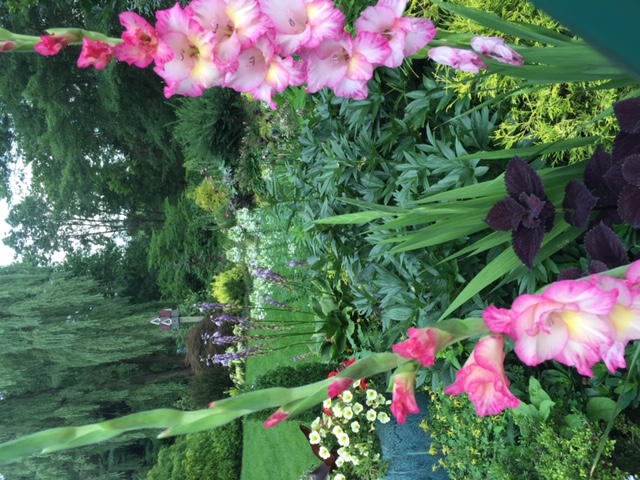This detailed photograph captures a lush, well-manicured garden brimming with a diverse array of vibrant flowers and foliage. In the foreground, tall plants with pink blossoms—likely hollyhocks or gladiolas—stand prominently, their petals ranging from dark pink to almost white. Interspersed among them are clusters of white flowers, some resembling morning glories with yellow centers, and elegant purple irises on sturdy stalks. A noticeable feature is a birdhouse with a red roof perched on a green post, nestled amid the foliage.

The mid-ground showcases a meticulously trimmed lawn, contrasting with the profusion of colors from the various blooms. To the left, a weeping willow gracefully arches its branches, and nearby deciduous trees add depth to the scene. The background is marked by an array of evergreen shrubs, purple bushes, and other large trees, including conifers, framing the garden setting. Despite some ambiguity about a potential stone feature or pond, the overall image is clear and vibrant, under a sky that appears either clear or lightly clouded, with sunlight subtly penetrating through the treetops. 

The photo radiates a serene, picturesque quality, capturing the natural beauty and tranquility of a lovingly tended garden.